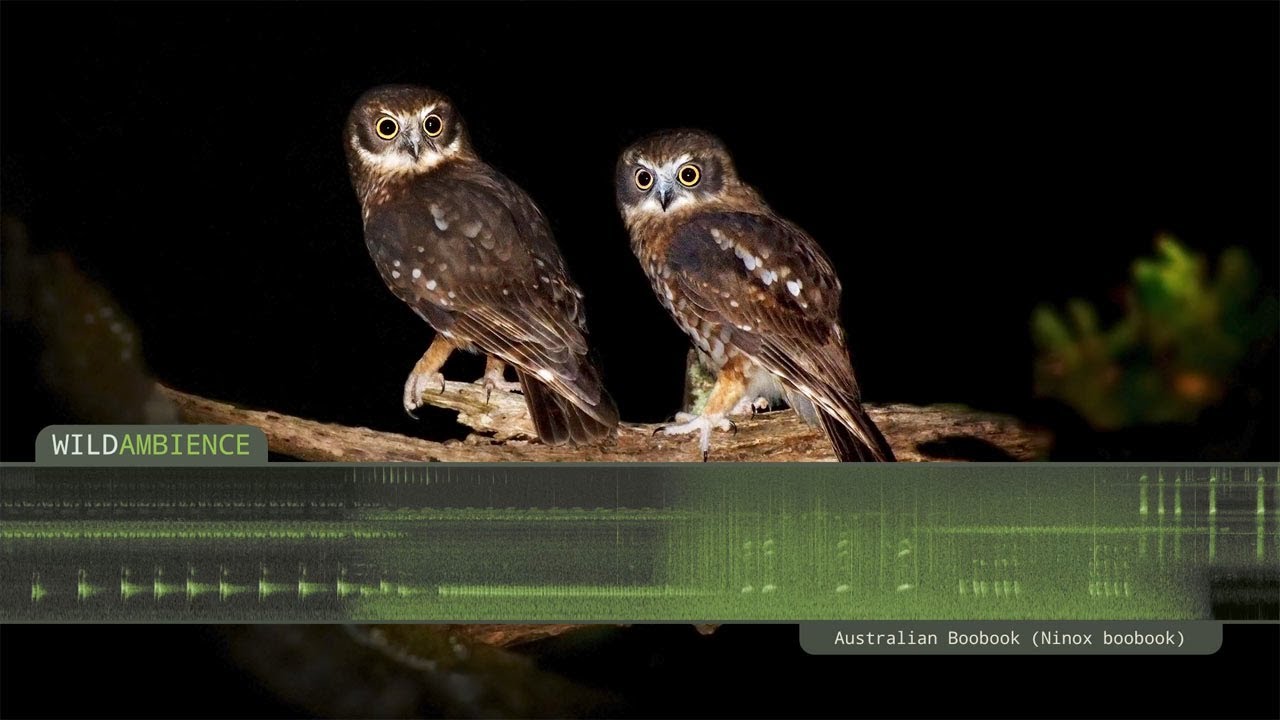The image features two brown owls with distinctive white markings around their necks, beaks, and eyes, perched on a weathered branch adorned with foliage on both sides. The owls, which have orange legs and black claws, are staring directly at the camera against a black background, suggesting it was taken at nighttime. A green banner at the bottom of the image reads "Wild Ambience" on the left side, indicating a sound display, while to the right, it states "Australian Boo Book (Ninox Boobook)" referencing the species of the owls. Beneath the banner, there is a spectrogram displaying the calls of the birds, adding an auditory element to the visual display. This setup implies that the image serves an educational or research purpose, possibly from a photography session or a project documenting these unique owls, which might be mates or part of the same family.